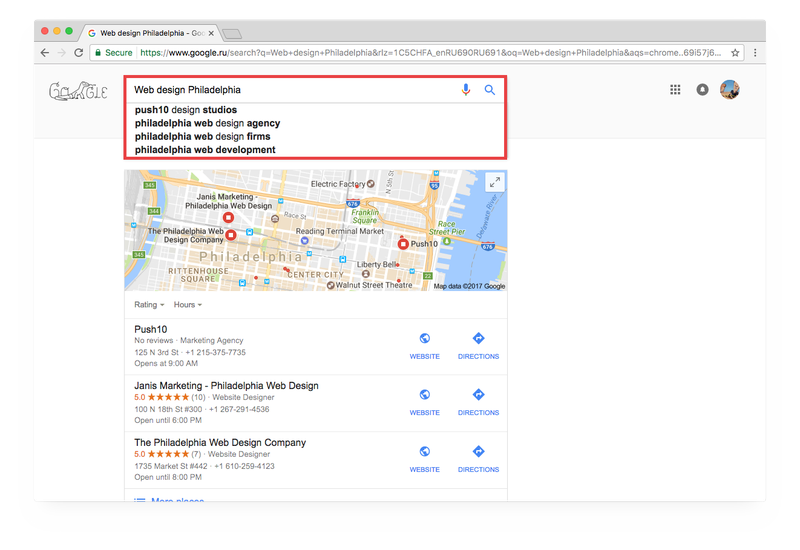The image is a detailed screenshot of a web browser accessing a Google search results page for "Web Design Philadelphia." At the top of the screen, the browser tab displays the text "Web Design Philadelphia." Directly below the tabs, a gray navigation bar indicates that a Google search has been conducted. The search query, "Web Design Philadelphia," is entered in the search bar.

Highlighted with a red rectangle beneath the search bar, several text-based search results are listed. These include "Push 10 Design Studios," "Philadelphia Web Design Agency," "Philadelphia Web Design Firms," and "Philadelphia Web Development."

Below these search result descriptions is an embedded map featuring several drop pins. The brown-colored areas indicate land, while a blue section to the far right represents water. 

Beneath the map, three specific business listings are displayed:
1. **Push 10**: To the right of this listing, options to visit the website or obtain directions are available.
2. **Janus Marketing, Philadelphia Web Design**: Similar options to visit the website or get directions are provided to the right of this listing.
3. **Philadelphia Web Design Company**: Likewise, this listing offers the choices of visiting the website or getting directions on the right.